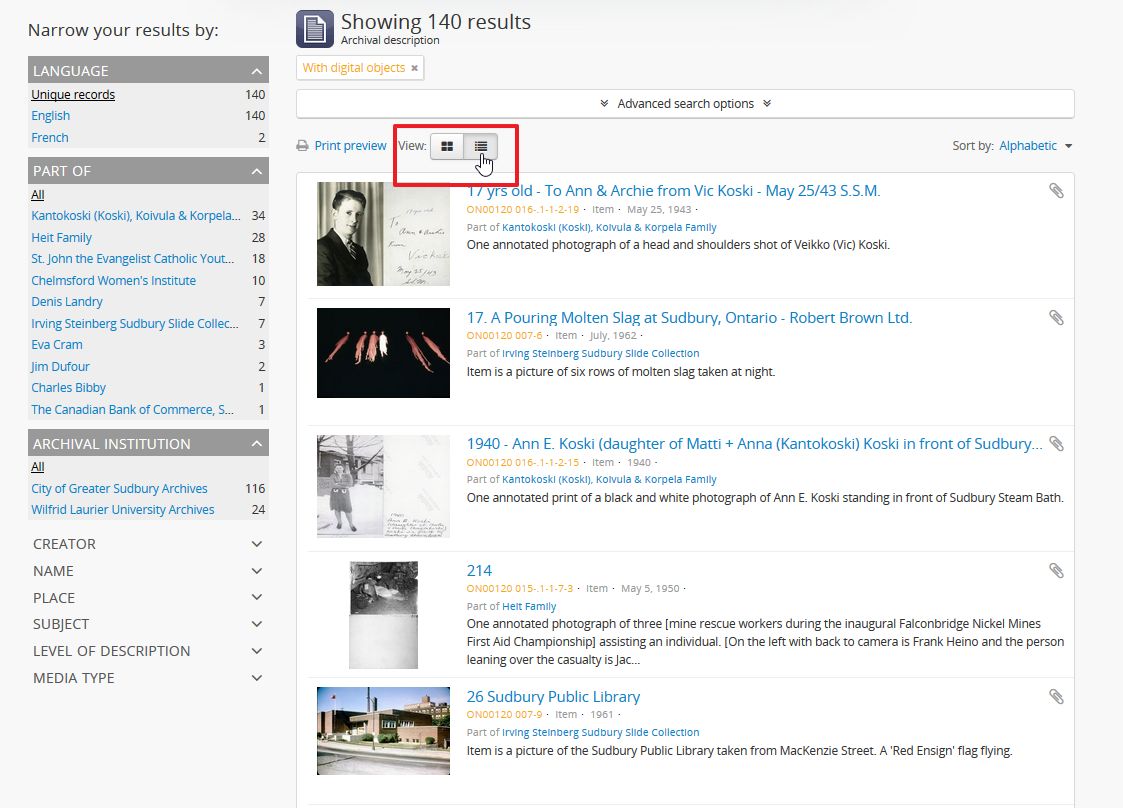This image appears to be a screenshot from a website featuring various filtering options and visual search results. The interface has a light gray background and contains a comprehensive sidebar and image display area. 

In the top-left corner, a dark gray header reads, "Narrow your results by." Directly below, various filter categories are listed in a structured manner. One prominent category, highlighted with a gray background, is labeled "Language" in white text. Under "Language," there are options for different languages such as English and French, each accompanied by specific numbers indicating the count of records.

Further down, another category titled "Part of" includes an "All" option with numerous blue text selections and their corresponding numbers. This is followed by the "Archival Institution" filter, also with a variety of selectable options. Additional categories listed below include "Creator," "Name," "Place," "Subject," "Level of Description," and "Media Type."

To the right of this filtering section, there is a collection of images and their corresponding captions. The images range from a man in a suit standing next to a whiteboard, to an all-black image portraying what appear to be aliens, a black-and-white photo of a woman in the snow, and an image of a building with a blue sky background. Each image is accompanied by descriptive text and selection numbers.

In the top right corner of each image section, there is a small thumbnail icon resembling a paperclip. A distinct red rectangle highlights an area with the word "View," accompanied by a small hand icon pointing to a selectable box, indicating an interactive element.